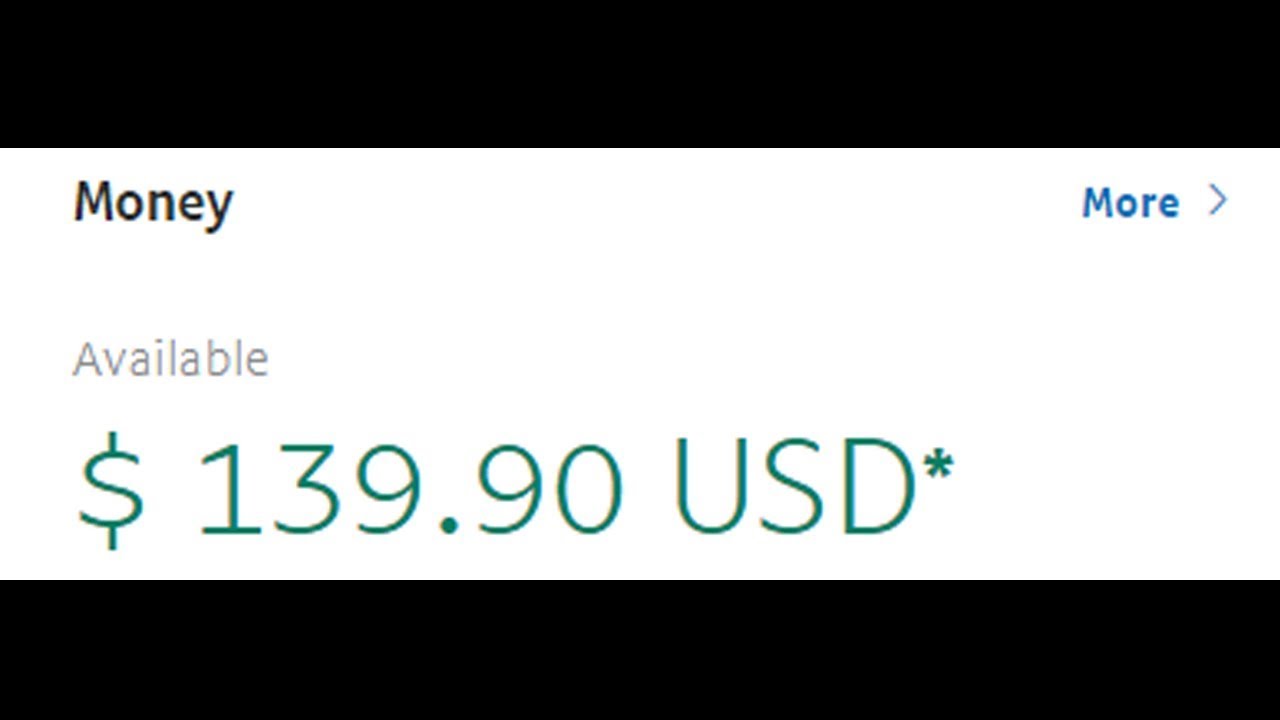Screenshot Description:

The image is a straightforward screenshot displaying the available balance in an unspecified account interface. The background is white, and the design is minimalistic, focusing solely on the balance information.

- **Top Left Corner:** A bold, black label simply reads "Money." Below it, in slightly smaller and semi-transparent grey text, it says "Available."
- **Balance Display:** Centrally positioned below the text labels, the available balance is highlighted in green characters: "$139.90 USD." Notably, there is an asterisk (*) immediately following "USD," though its exact purpose remains unclear.
- **Top Right Corner:** There is a clickable "More" button accompanied by an arrow, suggesting additional options or detailed information about the balance or transaction history could be accessed if clicked.

Overall, the image conveys a clear and focused snapshot of an account balance, possibly from a financial app like PayPal, though the specific application is not identifiable from the screenshot.